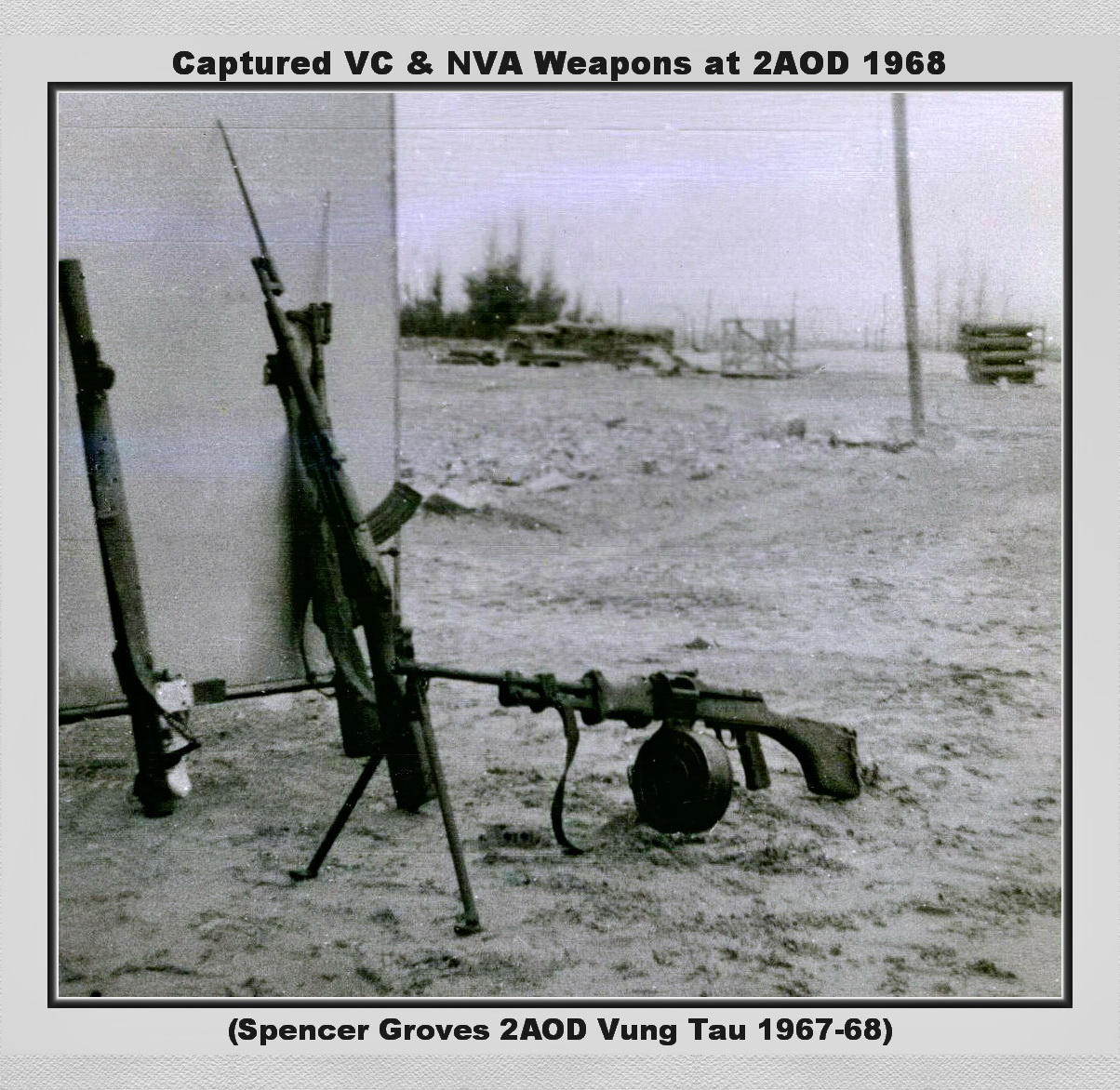This black and white photograph, bordered by a thin black and gray frame, captures a collection of captured VC and NVA weapons at 2AOD in 1968, as noted by the text printed at the top of the image. Below, a parenthetical caption reads "Spencer Groves, 2AOD, Vung Tau, 1967-68." The scene, slightly out of focus, appears to be outdoors in a field, with trees and military hardware visible in the background. On the right side, some pallet-like structures and a pole can be discerned. The center of the image prominently features a variety of weapons: three long rifles or machine guns are propped up against a wall, with two of them equipped with bayonets. Additionally, a machine gun with a bipod stand lies on the ground, showcasing a round chamber for bullets. Another weapon, possibly a handheld grenade launcher, is also present among the debris scattered across the field. The photograph effectively documents the remnants of combat gear, preserved in this moment of military history.